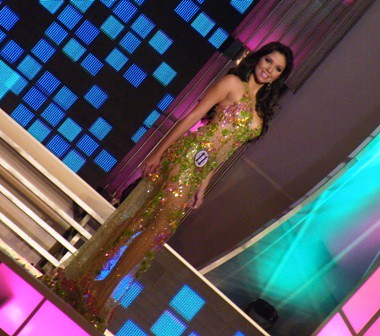The image showcases a model or pageant contestant, potentially from an event like Miss America or Miss Universe, confidently standing on a stage. Positioned centrally in the image, she is captured in a diagonal downward stance, smiling directly at the camera. She has dark brown or black hair and a darkish light skin tone, complementing her dazzling, glittery, and semi-sheer dress that features a vibrant blend of gold, green, and pink hues. This dress elegantly exposes her legs, emphasizing its fashionable and bold design. A small round card with the number 11 is affixed to her hip. 

The stage setting is illuminated by an array of neon and blue lights, contributing to a lively and dynamic atmosphere. Behind her, a set of tanned stairs, likely the path she descended, leads up to a backdrop embellished with an intricate array of shapes and patterns. These include dark blue and light blue squares, turquoise lines, and accents of neon pink. The entire scene, reminiscent of a high-energy catwalk or game show setting, is vividly colorful with a multitude of neon hues—green, light green, blues, whites, and grays—that enhance the model's striking appearance and the overall visual appeal.